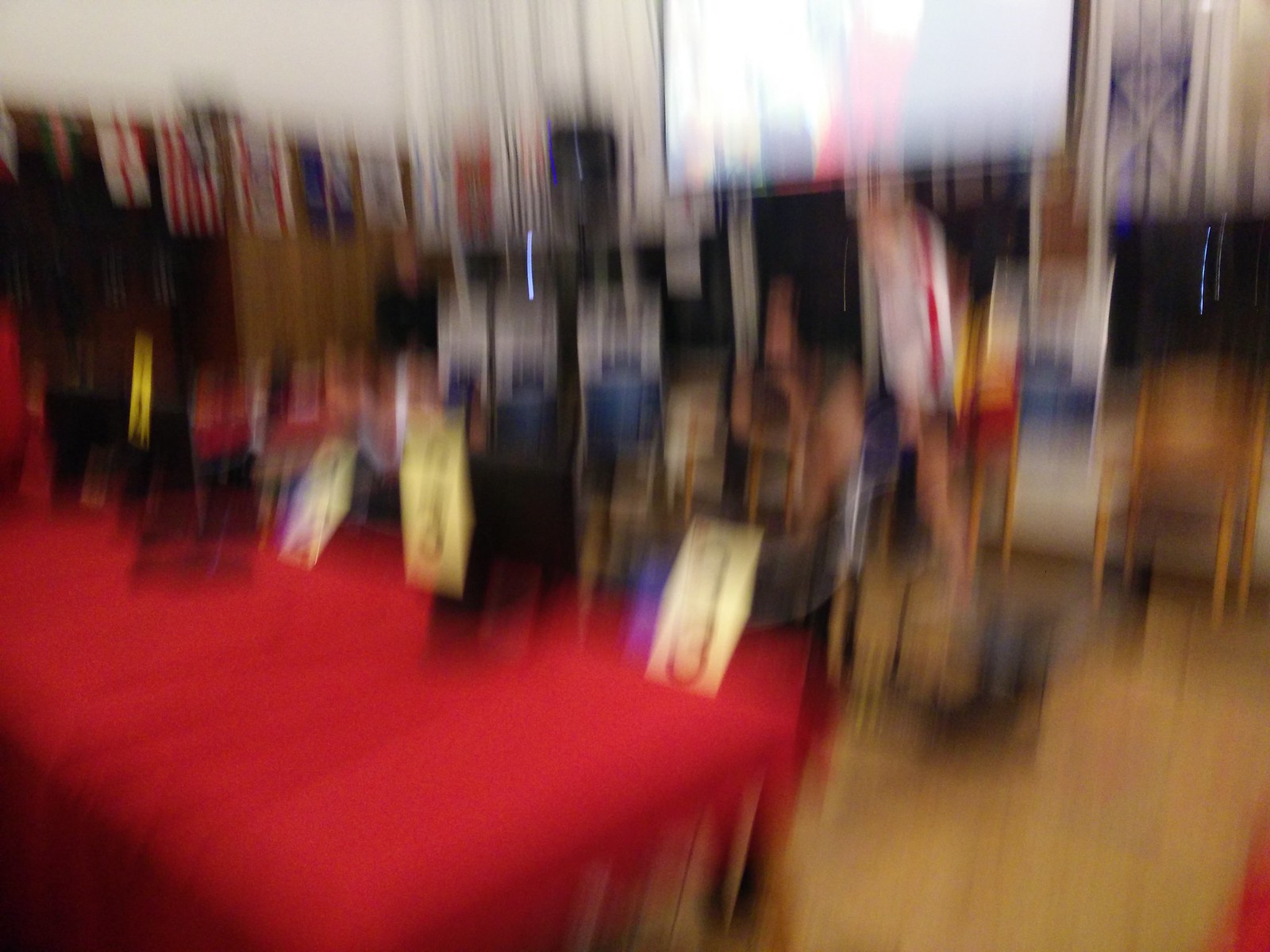The picture is very blurry, with a pronounced streaking effect that suggests movement occurred when it was taken. Despite the blur, it's evident that the photo depicts a room with a brown floor and various elements that are hard to discern clearly. Central to the image is a red table or altar positioned toward the front, bearing what seem to be rectangular, gold objects and possibly people's pictures. The background features a large projector screen on the wall, flanked by what appear to be flags or framed art. Several blue and white structures, leaning against the wall, are also visible amidst a lot of black shadows. The room has a few chairs scattered about and the overall lighting and blur cast a shadowy, elongated look on the items. The red table appears to sit on a raised platform, possibly covered with thick red material and bordered by a brown skirt, adding a sense of depth despite the blurriness.